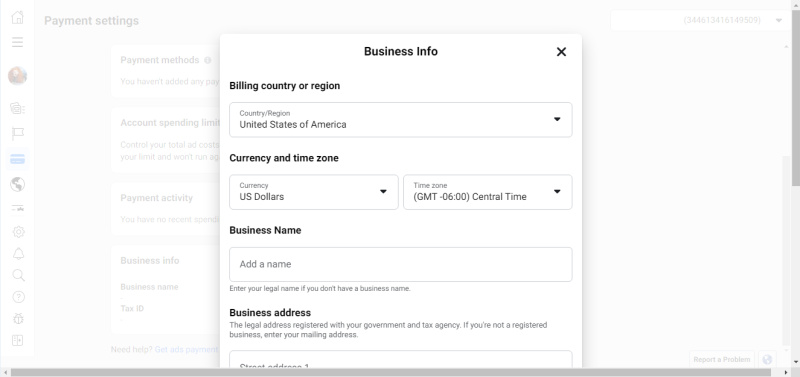The pop-up window displays a comprehensive form for entering business information. At the top of the form, a drop-down menu lists various options for selecting the billing country or region, which is currently set to the United States of America. Below this, there are sections for entering the currency and time zone, with the currency preset to US dollars and the time zone set to Central Time.

Further down, a field labeled "Business Name" is empty, accompanied by smaller text advising users to enter their legal name if no official business name exists. 

The next field requires the business address, specifically the legal address registered with the government and tax agency. If the user is not a registered business, they are instructed to provide their mailing address. 

Towards the bottom, the form details "Payment Settings," including sections for account spending, payment activity, and several icons on the left side, such as a globe, flag, search icon, alert symbol, and help button.

If users wish to exit this pop-up and return to their previous work, they can click the 'X' in the payment settings web area. The form is meticulously designed to ensure accurate business information collection, covering all necessary aspects from basic identification to specific legal and payment details.